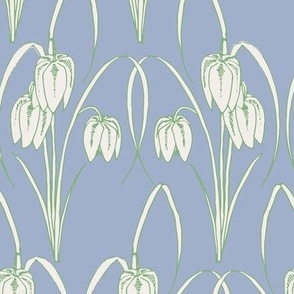The image is a square, digital print piece featuring a seamless pattern of white flowers with green borders and thin green stems, all set against a blue background that is slightly lighter in the lower left-hand corner. The flowers, which resemble tulips, hang downwards rather than standing upright. The pattern repeats across the image, giving it the appearance of a wallpaper design. The composition lacks any text, borders, or human elements, creating a simplistic and somewhat unappealing aesthetic often associated with bland home decor. The uniformity and repetitive nature of the pattern, combined with the dull color palette, suggest it could be used as a decorative background, although its visual appeal is limited.